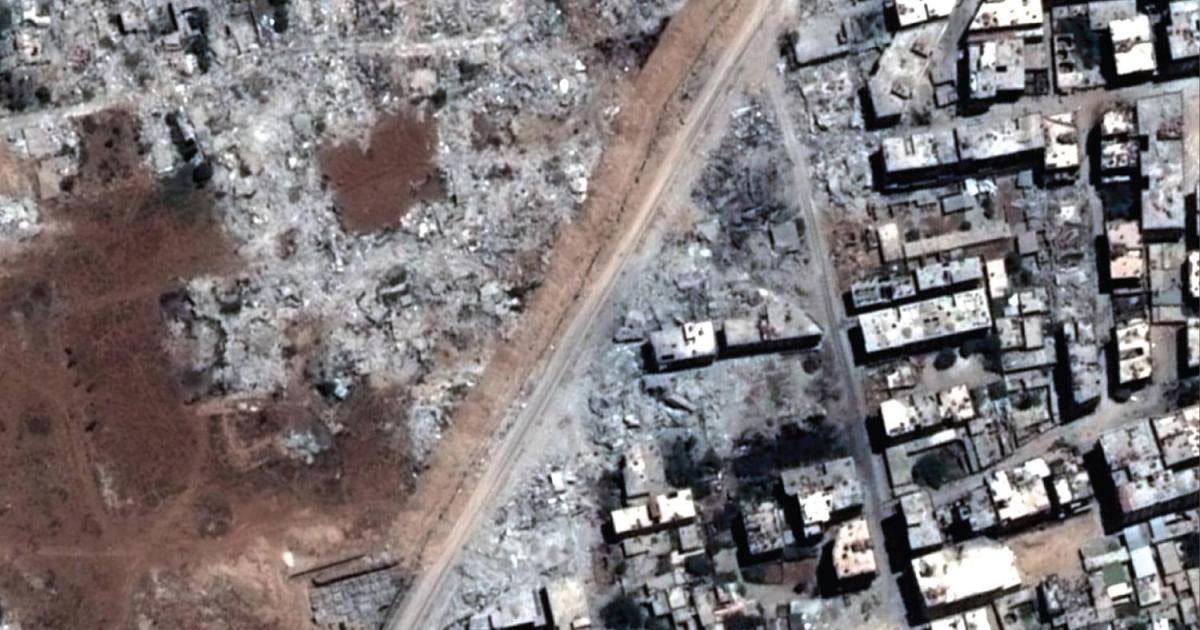This aerial view captures a landscape bisected by a diagonal trail that stretches from the lower left to the upper right of the image. The exact nature of the trail is uncertain; it could be a road or railroad tracks. To the left of this trail lies a sparsely populated area characterized by brown dirt and scattered, indistinct buildings, which seem to sit on ash-laden ground. The environment here appears to be heavily affected by something that has resulted in piles of ash, giving the area a desolate look, with little discernible structure and no vegetation. There is a square patch of brown amid the gray ash, possibly indicating some kind of land feature or a cleared area.

To the right of the trail, the scene transitions into a more densely populated area with numerous buildings and houses. These structures are larger and longer, suggesting they might include businesses and stores. However, these buildings also show signs of damage or burning, blending into the gray and white tones of the landscape. The lack of trees and the predominance of dirt and ash create a stark and bleak atmosphere across the entire scene.